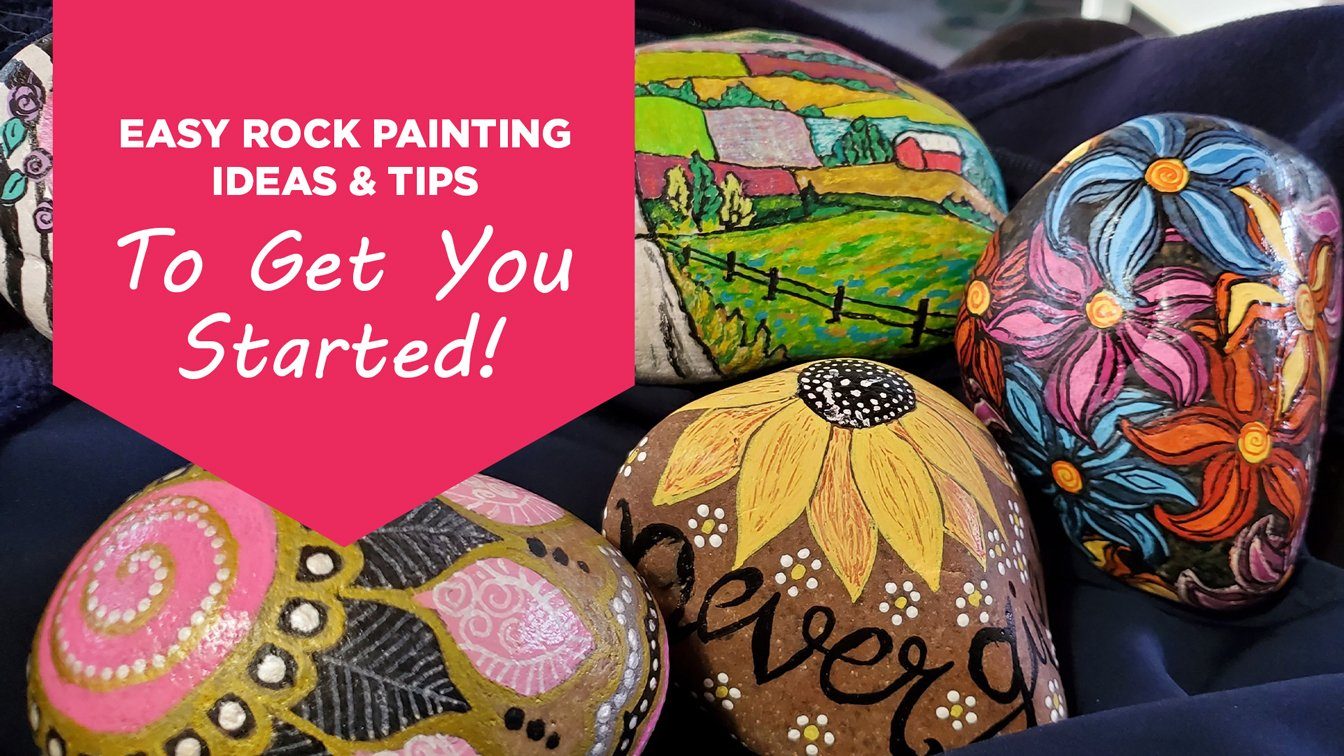This vibrant photograph showcases a collection of four medium-sized painted rocks, artfully arranged on a velvety cloth. A vibrant red, upside-down pentagon banner in the top left corner features the text "Easy Rock Painting Ideas and Tips to Get You Started!" in white font, with the phrase "to get you started" emphasized in larger letters. The first visible rock displays a charming barn scene set against a rustic backdrop. The second rock is adorned with an array of colorful flowers—blue, purple, orange—all with yellow buds. The third rock, painted with a motivational message "never give up" in black writing, features a large sunflower surrounded by delicate polka dot flowers. The final rock presents a meticulously detailed mandala design with a pink spiral pattern to the side. These captivating painted rocks each weigh between three to five pounds, offering substantial, real rocks rather than mere stones, poised to inspire rock painting enthusiasts.